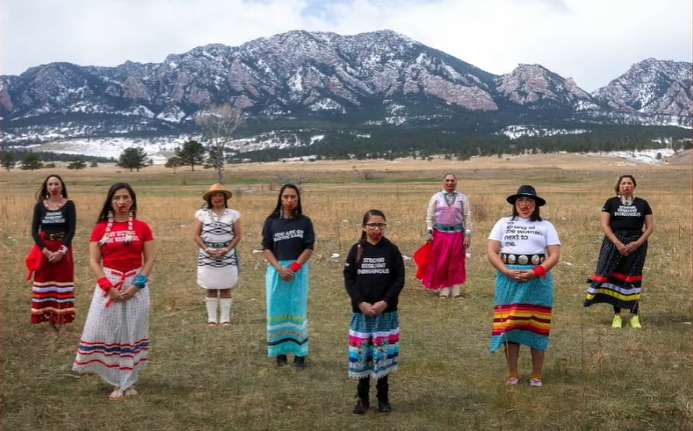In this photo, a group of Native American women and girls of varying ages stand in a zigzag formation around 2 meters apart in a green and yellow field with short grass. Behind them, a breathtaking vista of snowy mountains stretches across the horizon. The women and girls, eight in total, face the camera, their expressions highlighted by red handprints painted across their mouths. They are adorned in vibrant, traditional-style skirts featuring bright colors and multiple stripes along the lower hems, paired with a mix of modern t-shirts and hoodies. Some of the t-shirts bear unreadable text; one discernible word is "resilient." All but one of the women have their hands clasped in front of them, with the eldest woman having her hands by her sides. The scene suggests a poignant display of cultural pride and solidarity, possibly linked to a demonstration or protest.